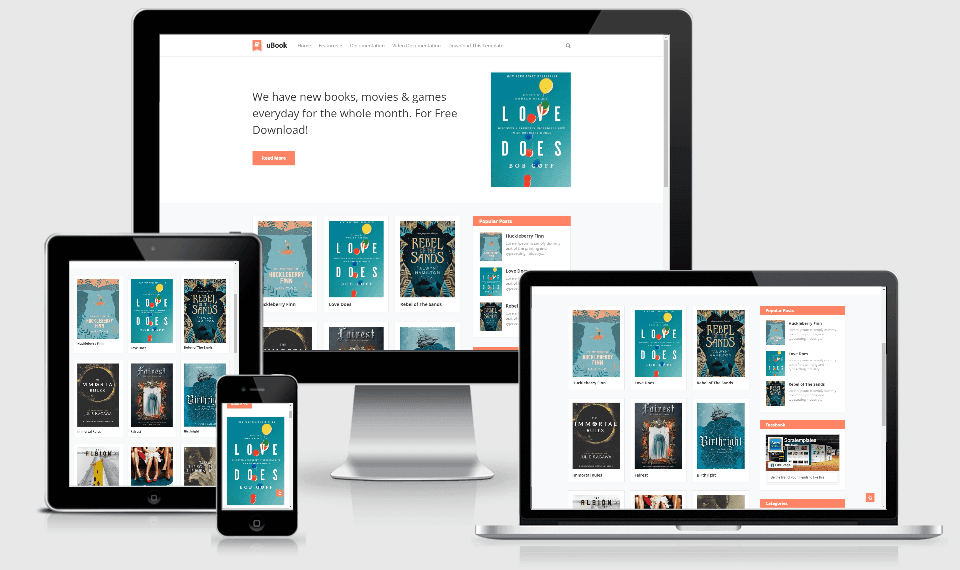The image is a mock-up of a responsive website designed to showcase its optimization across various devices. The website belongs to eBook, featuring a clean white background accented with light coral orange highlights. At the top of the site, there's a navigation menu alongside the eBook logo, which resembles a ribbon or the bent-over part of a bookmark, giving it the appearance of a hanging banner.

Below the logo, a prominent banner announces, "We have new books, movies, and games every day for the whole month for free download." A coral-colored rectangle with white text serves as the download button directly beneath this announcement.

The featured book is "Love Does," displayed against a sky background adorned with yellow, red, and blue balloons, where the yellow balloon is the most prominent at the top. Other visible books include updated cover versions of "Huckleberry Finn," "Love Does," and "Rebel of the Sands," along with additional titles that are partially cut off.

The website's layout is also depicted across multiple devices in the background, including a widescreen Mac monitor, an iPad, an iPhone, and an open MacBook, all set against a gray backdrop.